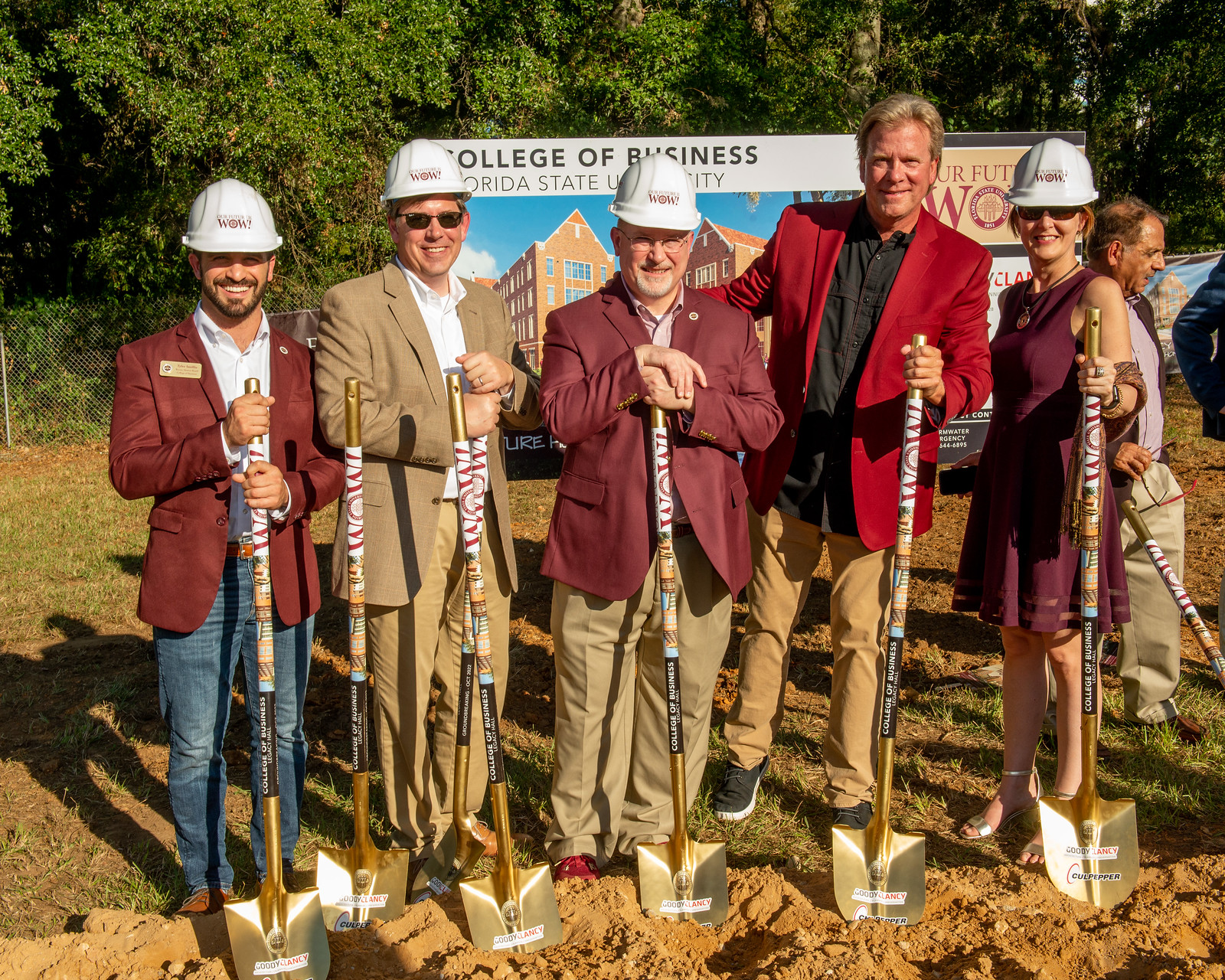The image depicts a groundbreaking ceremony for the College of Business at Florida State University, featuring a group of five individuals standing on a dirt field with wide smiles, posed to commemorate the event. Four men and one woman are lined up, each holding a golden shovel. The four men are wearing white construction helmets, adding a touch of formality and safety to the occasion, while the man on the far right, who is looking off to the side, does not wear a helmet. From left to right: the first man sports a red suit jacket, white shirt, blue jeans, and a helmet; the second man, in a tan suit with white shirt and tan pants, also wears a helmet and sunglasses; the central figure, a man clad in a red jacket, pink shirt, and khaki pants, completes the suited trio and wears a helmet. The fourth person, a man without a helmet, is in a red jacket, black shirt, and khaki pants, and has blonde hair. On the far right, a woman in a maroon dress and sunglasses holds her shovel, matching her colleagues in enthusiasm. Behind them, a bright, clear banner announces the Florida State University College of Business, surrounded by lush green trees, under a sunlit sky, emphasizing the bright and optimistic setting of this outdoor event.